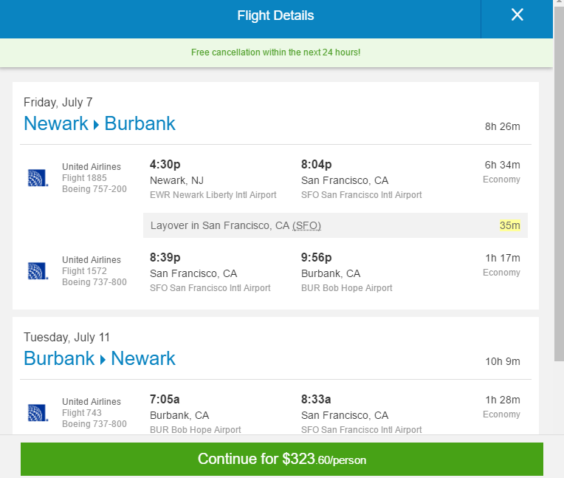A detailed webpage image is displayed, showing flight details within a blue box at the top. The box has a white 'X' on the right for closing the window. The main title states "Flight Details" and highlights that free cancellation is available within the next 24 hours.

For the outbound flight on Friday, July 7th, it outlines the journey from Newark to Burbank with United Airlines flight 430. This flight lands in San Francisco at 8:04 PM, after which there is a layover of 6 hours and 34 minutes. The journey from San Francisco to Burbank is on United Airlines flight 839, departing at 9:56 PM and lasting 1 hour and 17 minutes. Both segments are economy class.

For the return flight on Tuesday, July 11th, the details state a departure from Burbank to Newark. The flight is United Airlines 705, leaving Burbank's Bob Hope Airport at 8:33 AM and arriving in San Francisco International Airport after 1 hour and 28 minutes in economy class.

At the bottom of the image, there is a solid green bar indicating the option to "Continue" for $323.60 per person. This bar suggests that users can proceed by clicking to potentially select or modify their flight for a slightly different fare.